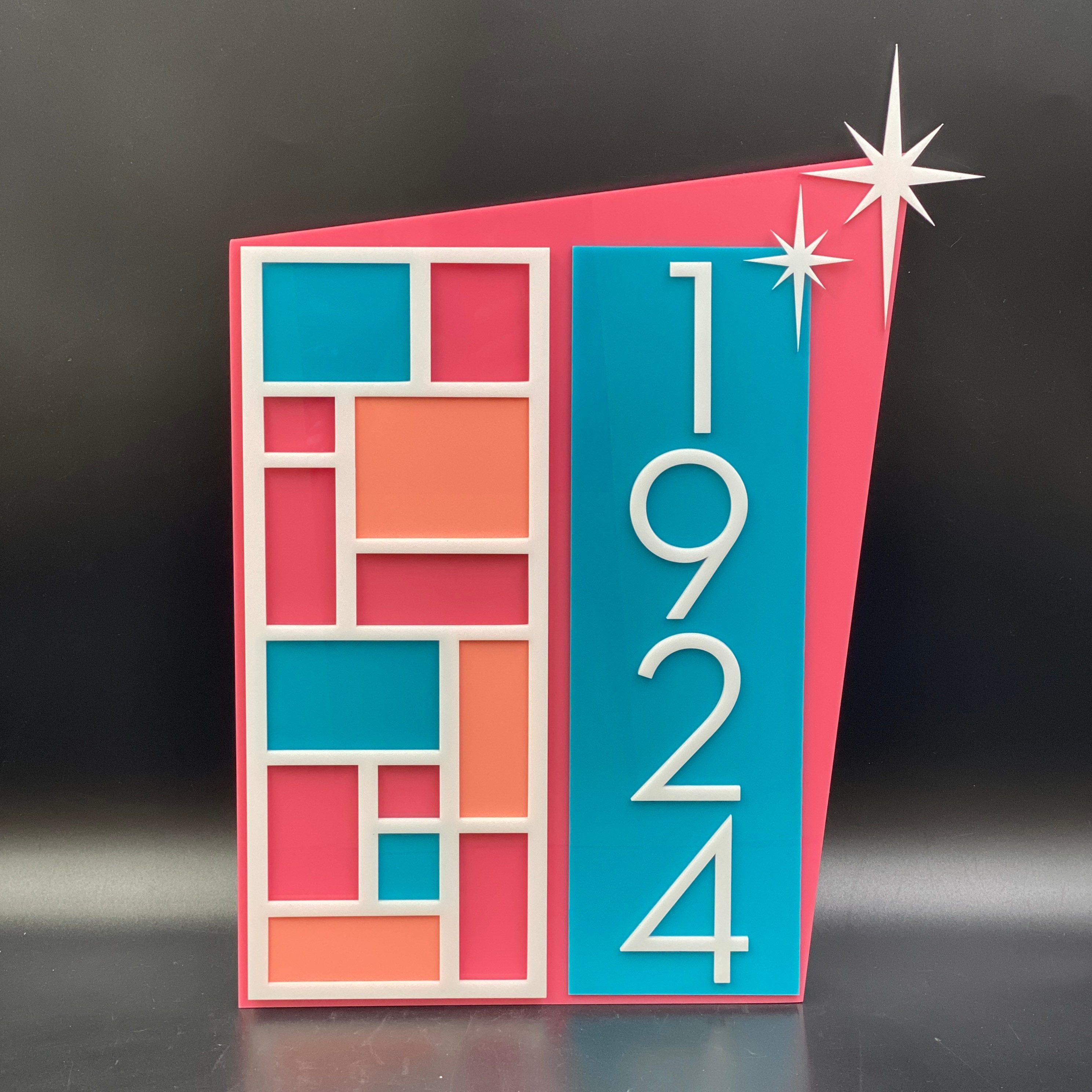The image showcases a 3D address sign that resembles a championship emblem, characterized by a flat bottom and left side, with the right side slanted upward and the top also slanting upward. The right corner prominently features a large white star with spiky rays. The sign's main body is pink, containing two distinct sections. On the left is a white rectangular frame embedded into the pink background, which houses multiple smaller rectangles in various colors such as blue, pink, and peach, separated by white lines. On the right side of the sign, there is a tall, vertical blue plate with the year "1924" engraved in white, and a smaller white star positioned in its upper right corner. The entire address sign has an abstract, artistic design, resembling a card or a yearbook cover set against a black surface.